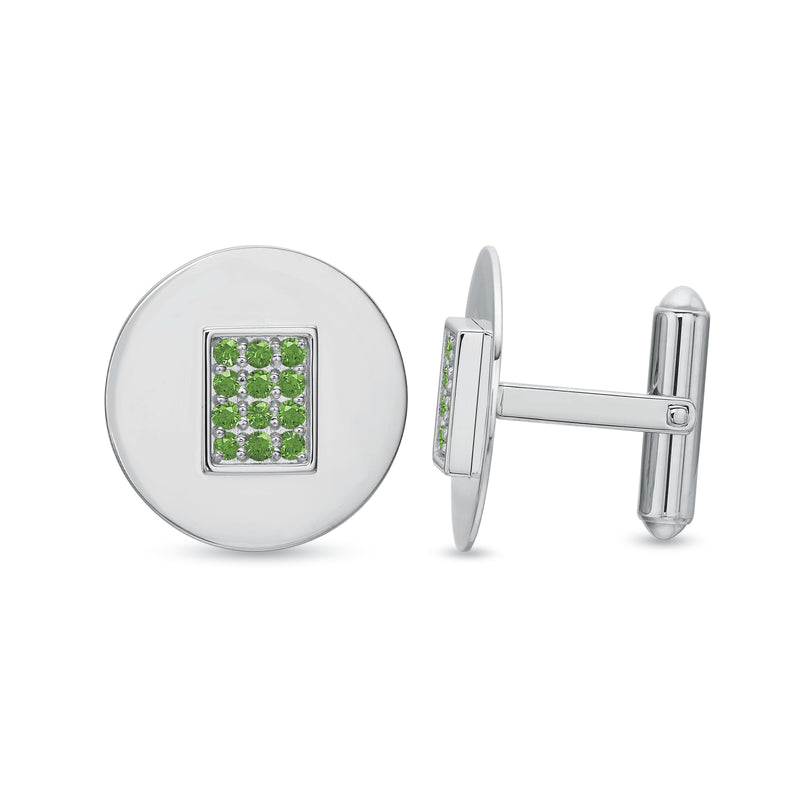The product image showcases a pair of men's cufflinks with a solid white background, ensuring the focus remains solely on the cufflinks. The image displays two views: a side profile and a head-on view highlighting the circular face of the cufflinks. Crafted from a silver-toned metal, the cufflinks feature a distinctive design on their round heads, which includes a raised square in the center. This central square houses a grid of twelve green gemstones, arranged in a four-by-three pattern, reminiscent of emeralds. The cufflinks are held together by a cylindrical bar extending from the back of the circular face, connecting to a smaller bar that likely serves as the fastening mechanism. The meticulous arrangement of the green gems and the sleek, shiny metal finish contribute to the cufflinks' elegant and sophisticated appearance.